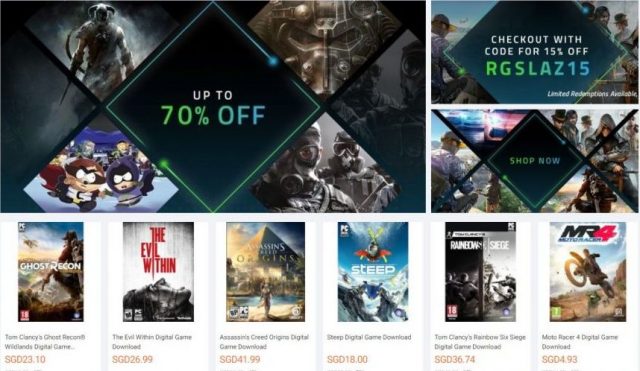The rectangular promotional image, oriented with its longer side stretching horizontally, appears to be tailored for gaming enthusiasts. The main layout is divided into a collage-like format, bordered by distinct white lines that separate various sections of the content.

Occupying the upper left portion, the largest segment showcases multiple gaming characters arranged in a diamond-like grid pattern. This segment prominently features a central text that offers "Up to 70% off," enticing potential buyers with significant discounts. Adjacent to this, a smaller banner on the upper right corner promotes an additional offer, stating "Check out with code for 15% off."

Just below the top section, another area continues the diamond-themed character display. At its core, a bold directive encourages viewers to "Shop Now," highlighting the urgency and appeal of the ongoing promotions.

The bottom third of the image is dedicated to displaying six distinct game titles, each with its own price tag. The prices listed are in dual formats, showing both SGD26.99 and $41.99, suggesting international pricing options. These game titles are likely popular selections, aiming to draw immediate interest from the viewers.

Overall, the image serves as a vibrant and detailed announcement for a sale, combining attractive discounts and specific call-to-action prompts to engage the target audience.